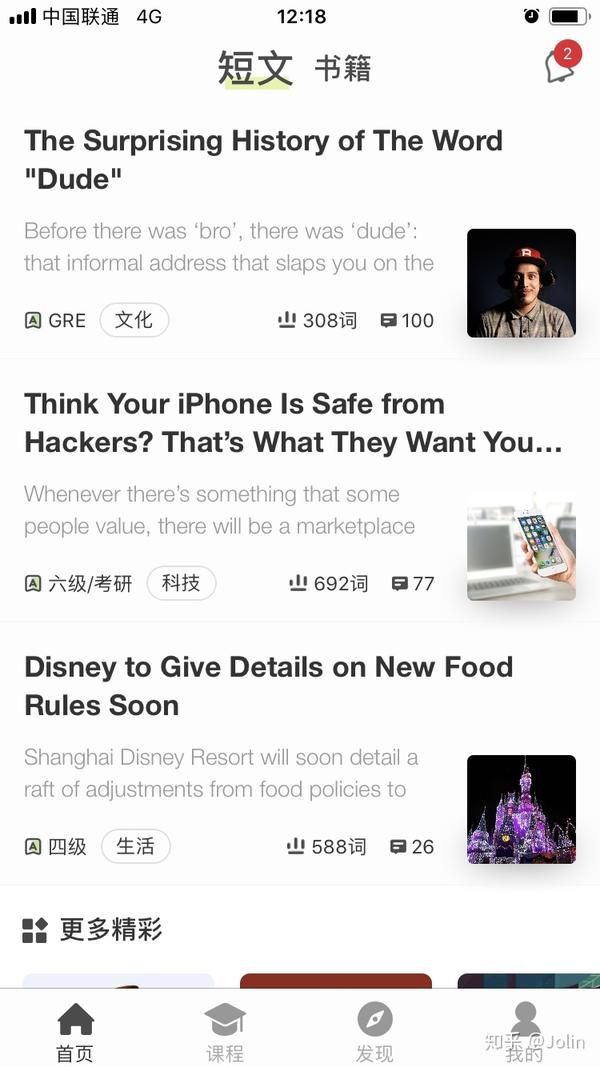In the image, we see a smartphone screen displaying various articles, indicated by the "4G" symbol on the top status bar. The text appears to be in an East Asian language, potentially Japanese or Chinese, given the stylistic script. At the top left corner, the Wi-Fi symbol is visible, confirming the device's internet connectivity. The time is prominently displayed at the top center, reading 12:18. On the top right corner, there are icons for battery life and an alarm clock.

The main article headline is highlighted in quotation marks, reading "The Surprising History of the Word 'Dude'." Below this, a subheading states, "Before there was bro, there was dude, that informal address that slaps you on the..." with the text trailing off. Accompanying this headline is an image of a smiling man wearing a red hat with an "R" on it and a beige button-up shirt.

Further down, several other article headlines are partially visible. The second headline starts with "Think Your iPhone is Safe from Hackers" before trailing off. Next to this headline, there is an image of an iPhone. 

The third visible article headline reads, "Disney to Give Details on New Food Rules Soon," accompanied by an image of a brightly lit Disney castle at night, glowing in purple, gold, and white lights.

Beneath these headlines, additional symbols and characters in the respective language indicate various metrics like the number of comments and views, though the specific details are not fully readable.